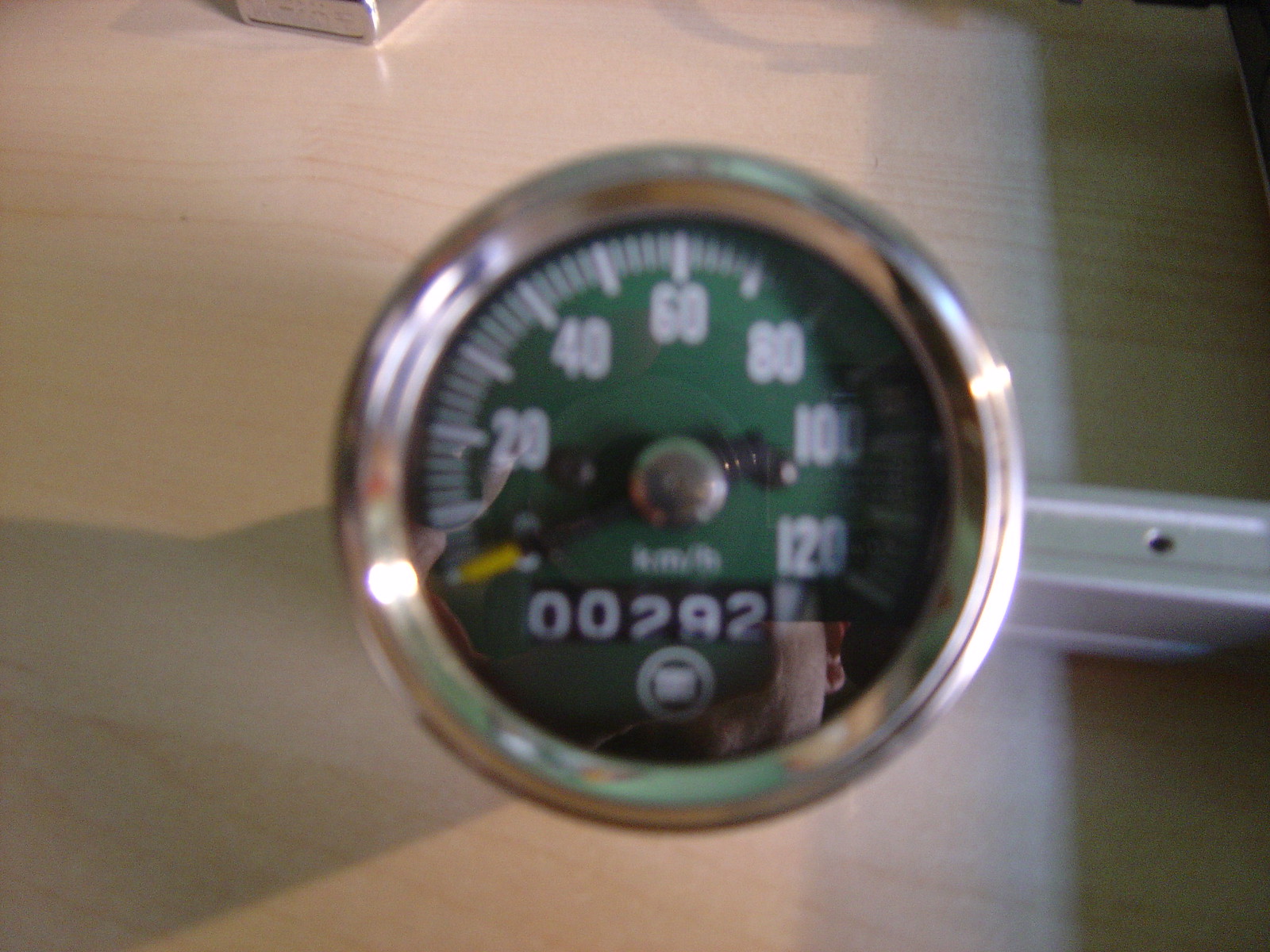The image captures a blurry photograph of a gauge resting on a light brownish-white wooden surface with a prominent horizontal grain pattern. The gauge, positioned too close to the camera, dominates the frame, making its details slightly unclear. It features a circular metal rim and a face with a dark green background. Encircling the gauge are white numerical markings in increments of 20, ranging from 20 up to 120. The gauge's dial is pointed at zero. At the bottom of the gauge face, a rolling numeric counter displays the number 00282. The glass of the gauge reflects the lower part of a man's face. Shadows cast on the wooden surface add depth to the image. Additionally, a stick extends from the right-hand side of the gauge.